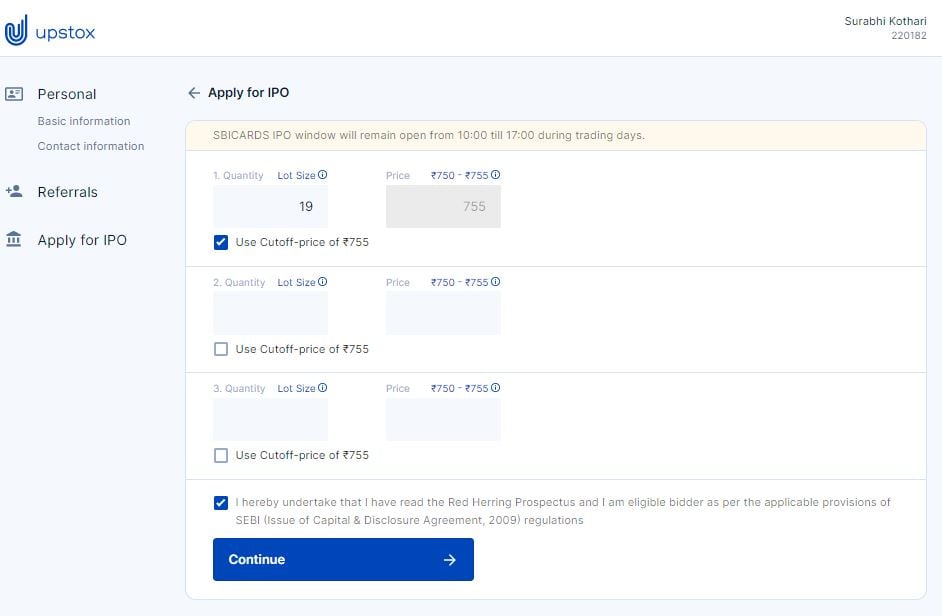Screenshot of the Upstox application interface displaying IPO application details for SBI Cards. At the top, the interface features the title "upstox" in lowercase letters. In the top-right corner, the user information "Surabhi Kothari 220182" is visible. The screen navigates through sections labeled "Personal," "Basic Information," "Contact Information," "Referrals," and "Apply for IPO."

An arrow pointing to the left is labeled "Apply for IPO." A notification states, "SBI Cards IPO window will remain open from 10 to 17 hours during trading days." Below, details of the IPO offering are listed: Quantity, Lot Size of 19, and Price ranging from 750 to 755 rupees, with the recommendation to use the cutoff price of 755 rupees, which is pre-checked. The same set of information is repeated for three entries.

At the bottom, a checked acknowledgment box contains the declaration: "I hereby undertake that I have read the Red Herring Prospectus and I am an eligible bidder as per the applicable provisions of SEBI Issue of Capital and Disclosure Agreement 2009 regulations." 

A blue rectangle with white interior text labeled "Continue" and featuring a right-pointing white arrow completes the interface. The image contains only textual elements and interface graphics, with no photographic content, people, animals, plants, or other natural elements.